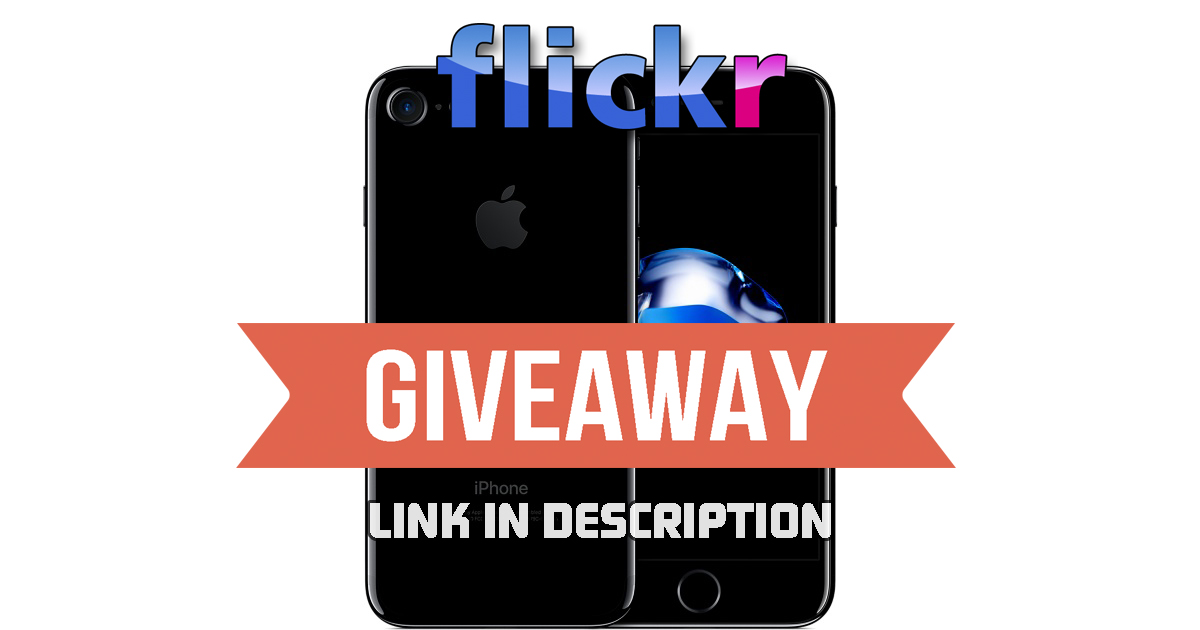The image features a simple, almost invisible white background displaying two views of a black Apple iPhone. On the left side, the back of the phone showcases a dark gray Apple logo and the word "iPhone." On the right side, the front of the phone features a blue and white 3D graphic on the screen, with a small home button at the bottom. Positioned at the top of the image, the Flickr logo is prominently displayed with 'Flickr' in blue and pink, where the 'R' transitions from a darker to lighter red. Below this, an orange-red banner with white text reads "Giveaway," followed by "Link in Description" in smaller white capital letters. The combination of these elements suggests this image is promoting an iPhone giveaway, potentially sponsored by Flickr.